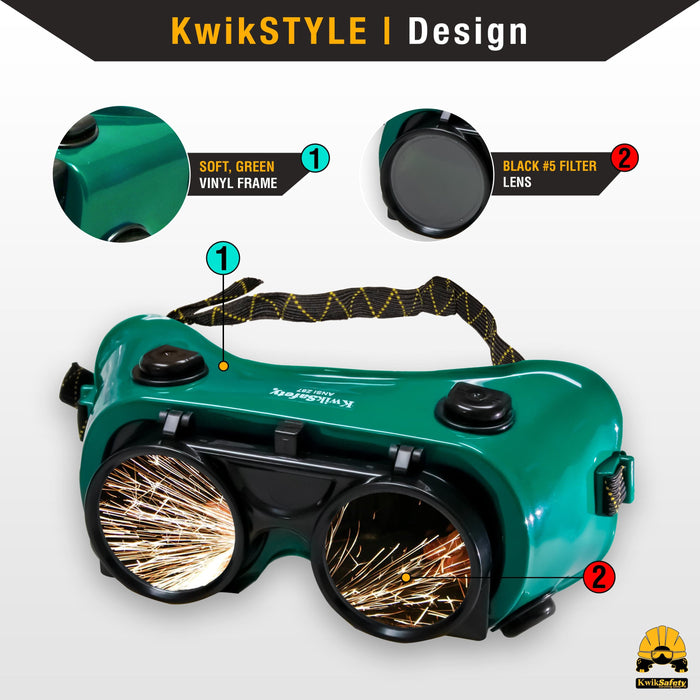The image is an advertisement for Kiewik Style safety goggles, designed for tasks like welding or sanding metal. The photo prominently features green plastic goggles with soft green vinyl frame, ensuring comfort for the wearer. The goggles include black number five filter lenses to protect the user's eyes from sparks, which can be seen reflected in the lenses, indicating their use in metalworking. A black head strap with yellow stitching secures the goggles in place. At the top of the advertisement, "Kiewik Style" is displayed, paired with a yellow horizontal divider labeled "Design." Two close-up features of the goggles are highlighted in an infographic: the soft green vinyl frame and the black number five filter lenses, enhancing their safety profile.